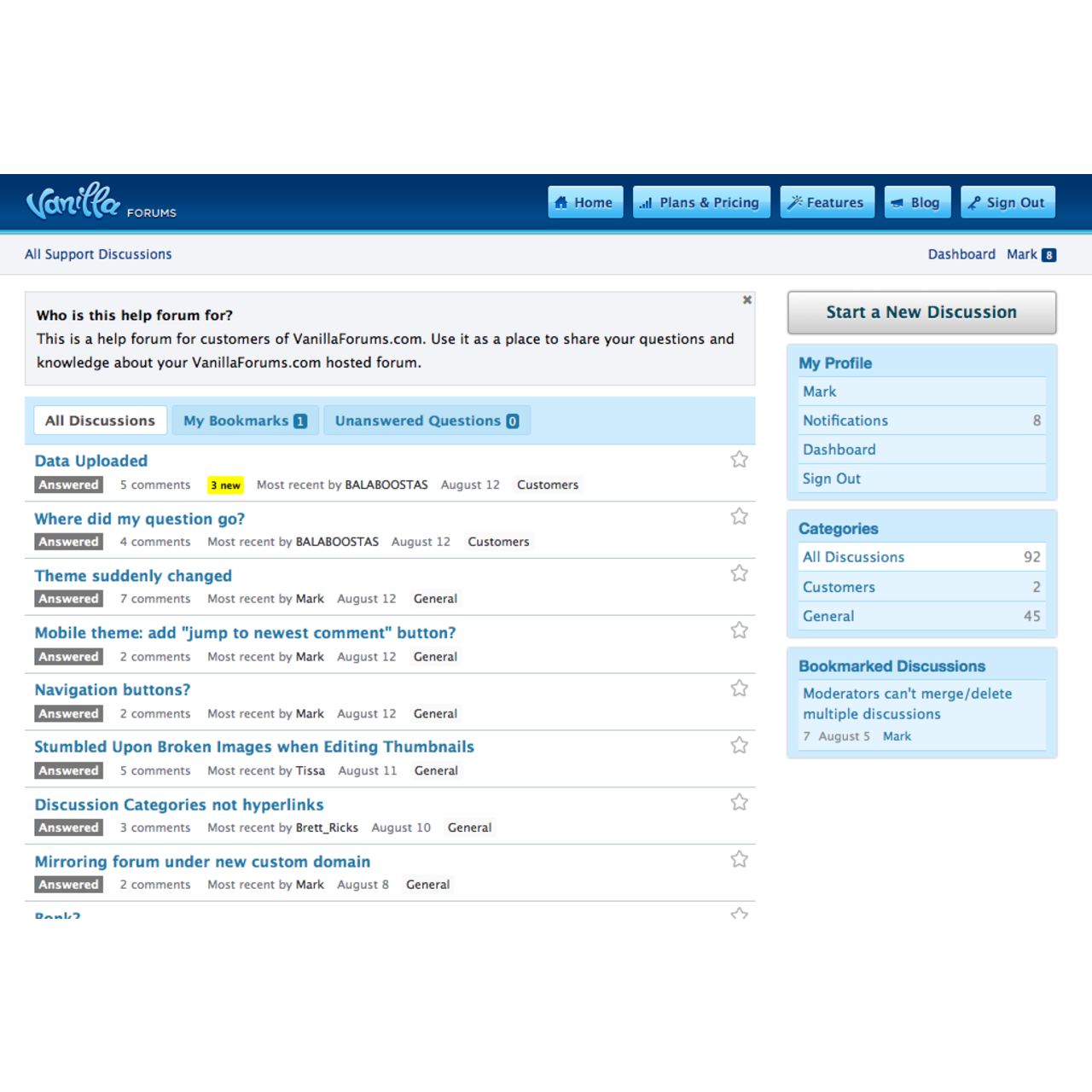**Detailed Caption:**

This screenshot captures the interface of the Vanilla Forms website. Prominently featured at the top left is the "Vanilla" logo, with the text "Vanilla Forms" beneath it. To the top right, a navigation menu is displayed, listing options from left to right: "Home," "Plans and Pricing," "Features," "Blog," and "Sign Out." Below the logo, the header "All Support Discussions" is visible, indicating the purpose of the page.

The main content area is dedicated to a series of support discussions for VanillaForms.com customers. A clear introductory message reads: "Who is this Help Form for?" followed by a description explaining that this is a help forum for VanillaForms.com customers to share questions and knowledge about their hosted forms.

A list of discussion titles occupies the central part of the screenshot. Topics include:
1. Data Uploaded
2. Where Did My Question Go
3. Theme Suddenly Changed
4. Mobile Theme Ad Jumped to Newest Comment Button
5. Navigation Buttons
6. Stumbled Upon Broken Images When Editing Thumbnails
7. Discussion Categories and Not Hyperlinks
8. Mirroring Form Under New Custom Domain

One specific discussion, "Data Uploaded," is highlighted in yellow, displaying additional details. It indicates there are five comments in this discussion thread, with three being new. This highlighted part suggests real-time updates for the comments section, helping users track new activity efficiently.